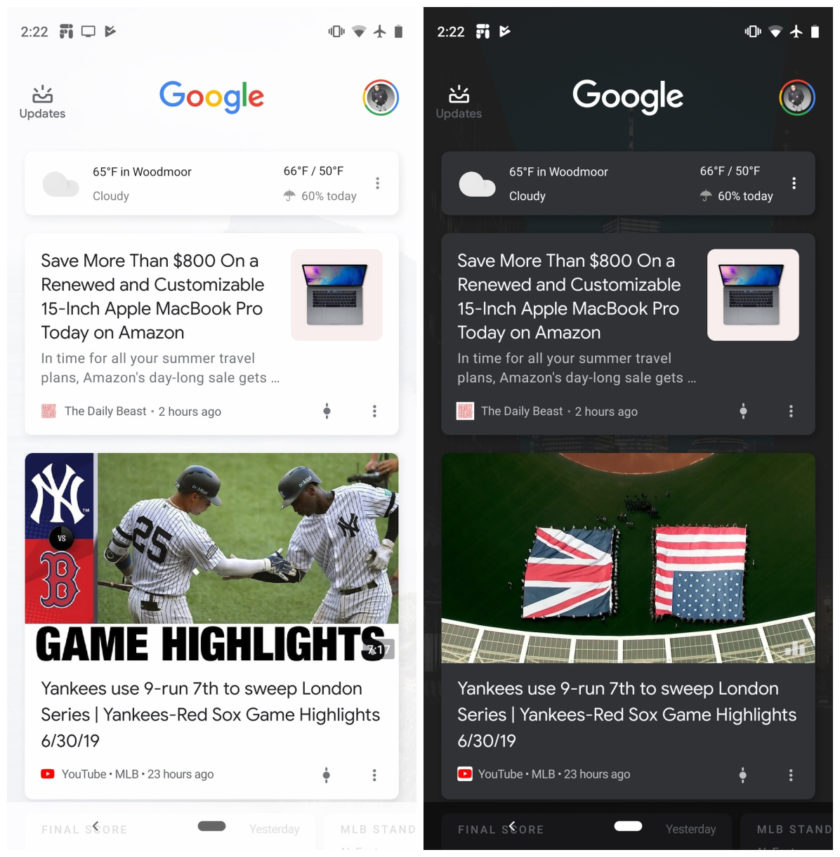This image showcases two screenshots taken from a cell phone, aligning side by side. Both screenshots are from different modes of the same interface—likely a mobile web browser or an application. 

The screenshot on the left features a predominantly white background. At the top, "Google" is prominently displayed in its standard colorful logo. Directly beneath, the weather information indicates it is 65 degrees in Widmore and cloudy, with a high of 66 degrees and a low of 50 degrees. A small umbrella icon signifies a 60% chance of rain. 

Further down, the left screenshot displays a promotional banner in white, advertising over $800 savings on a renewed, customizable 15-inch Apple MacBook Pro available on Amazon. Below this, a section titled "Game Highlights" discusses recent updates about the Yankees.

In contrast, the screenshot on the right presents the same information but in a dark mode interface with a black background. Here, the "Google" logo is rendered in white. The weather information, including temperature, high and low predictions, and the rain forecast, mirrors the left screenshot. Similarly, an advertisement for the discounted Apple MacBook Pro appears, albeit in a dark-themed layout. Unlike the left screenshot, the section labeled "Game Highlights" on the right features two sets of flags instead of discussing the Yankees.

Overall, the image compares the same content being displayed in both light and dark modes on a mobile device.